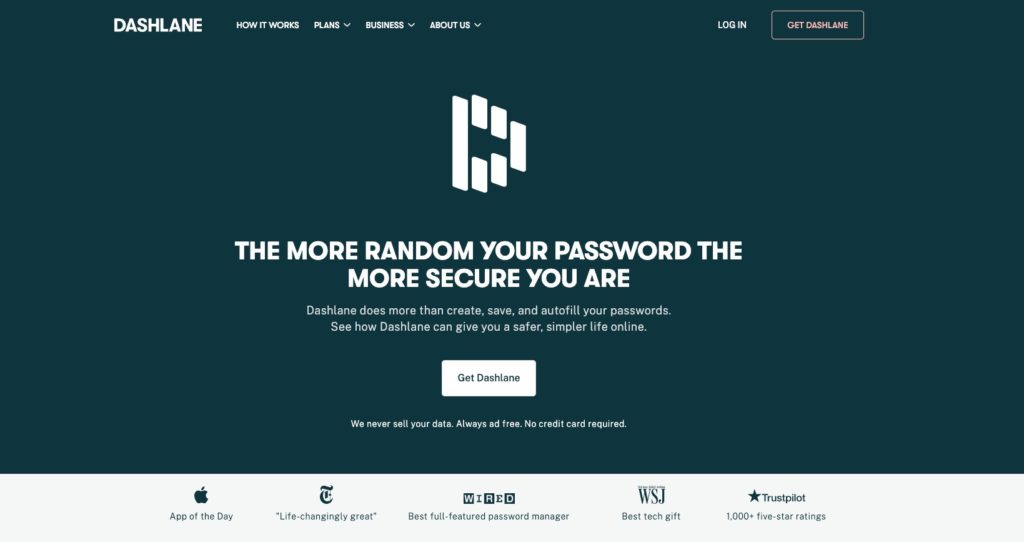The image appears to be a screenshot from the Dashlane website featuring a detailed layout of its homepage. In the upper left corner, "DASHLANE" is prominently displayed in white, bold, capitalized text. To the right of the logo are navigation links labeled "How It Works," "Plans," "Business," and "About Us," each accompanied by a drop-down menu arrow. On the far right, options for "Login" and "Get Dashlane" are visible, with "Get Dashlane" highlighted in a distinctive pinkish text.

At the center of the page, a stylized "D" logo, composed of various rectangular shapes and text boxes, captures attention. Adjacent to the logo is a message emphasizing the importance of secure passwords: "The more random your password, the more secure you are." Below this, it states that Dashlane offers more than just password creation, saving, and autofilling; it provides a safer and simpler online life. Below this message, a prominent white button labeled "Get Dashlane" invites users to engage further.

The lower section of the page reassures users with statements like "We never sell your data," "Always ad-free," and "No credit card required," all set against a dark blue background. At the very bottom, accolades from reputable sources are displayed: "App of the Day" with an Apple logo, "Life-changingly great" from The New York Times, "Best full-featured password manager" from Wired, "Best tech gift" from The Wall Street Journal, and "1,000+ five-star ratings" from Trustpilot.